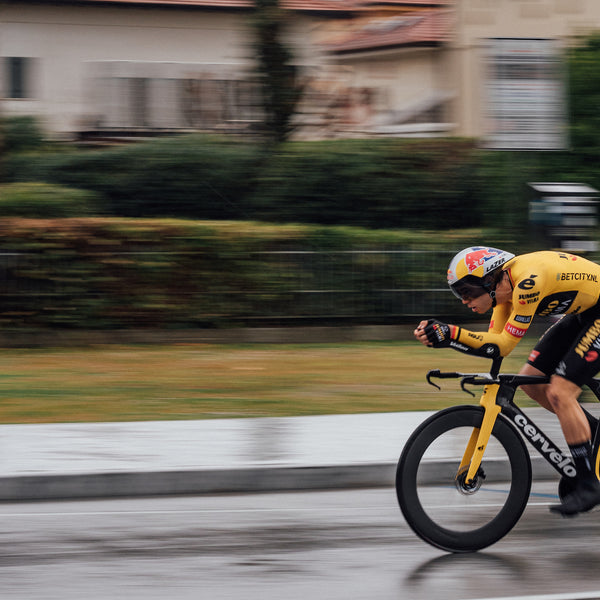The image is an intentionally blurred photograph with a clear focus on a cyclist in the right-hand foreground. The cyclist, who appears to be participating in a race, is riding a yellow and black Cervelo bike with thick tires. He is dressed in a yellow jersey adorned with various stamps, black cycling shorts, and socks. His helmet is detailed with white, red, blue, and yellow colors and features a black visor. The cyclist’s posture is aerodynamic, with his elbows resting on specialized handlebars that have forward-facing hooks. His head is down, displaying a look of determination. The blurred background suggests a residential area with a grey road, pavement, grass, a hedge, trees, and indistinct buildings.